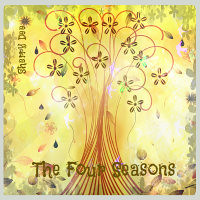The image presents an abstract illustration with a pale yellow background, resembling a tiny stamp. In the center, there is an artistic portrayal of a tree made of brownish lines that curl at the top. Surrounding the tree are a few dark petals or floral designs, suggesting falling leaves. The tree itself is sparsely populated, lacking a full canopy of leaves. In dark green, stylized, nature-inspired font, the text "happy day" appears on the upper left, although it is somewhat ambiguous. At the bottom, the phrase "the four seasons" is inscribed, though due to the small size, the exact wording is challenging to discern.